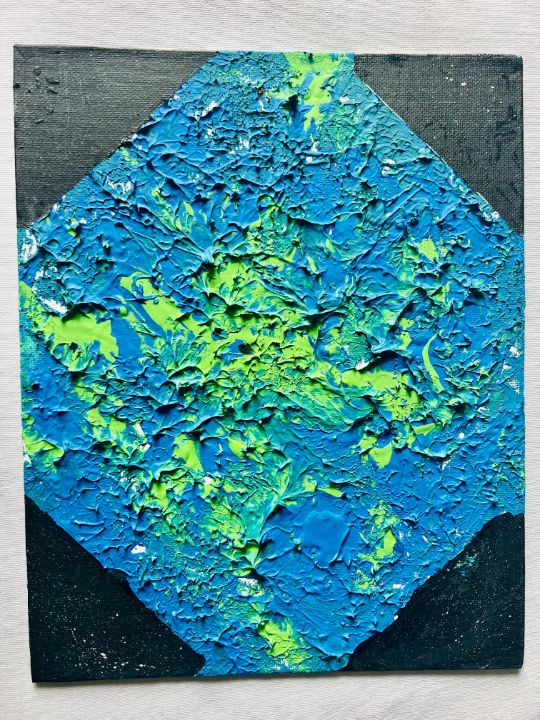The image depicts a striking piece of potential art, prominently featuring a vertical rectangular canvas. Dominating the composition is a distinctive square at the center, tilted on its angles, which extends beyond the canvas's top and sides. This focal square is lavishly coated with heavily applied, textured paint in vibrant hues—primarily a rich blue interspersed with chartreuse green and bright yellow. The texture in the square is palpable, with visible peaks and gobs of paint creating a dynamic, tactile surface. Within this textured mass, the chartreuse and yellow predominantly occupy the center, extending towards the left and bottom, with a notable splash at the top.

Surrounding the central square, the background appears as a dark, near-black blue, applied in a flat, smooth manner with occasional intentional gaps that expose a speckled or flecked underlayer. This contrast in texture between the smooth, almost flat backdrop and the thick, chaotic central square enhances the piece's visual impact. The overall composition and meticulous layering of colors suggest a carefully crafted artistic endeavor, possibly painted on a surface resembling light slate gray wood or stone. The artwork hangs in a white, textured-wall setting, emphasizing the piece's depth and thoughtful complexity.